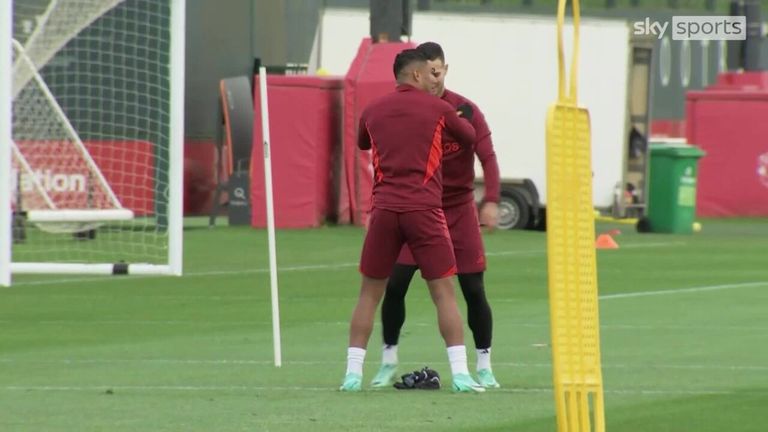This color photograph captures two male soccer players engaged in what appears to be calisthenic exercises on a lush green soccer field, with both players dressed in maroon uniforms accented by orange highlights. The player in the foreground has his back to the camera, wearing short white socks and green soccer cleats. Facing him is the second player, distinguished by his long black leggings paired with white socks and also wearing green cleats. Both players sport short black hair. The scene includes part of a white soccer goal with netting visible on the left, though partially cropped out. In the background, there are various elements including red pads, a green garbage can, and a white trailer. The Sky Sports watermark is prominently displayed in translucent white in the upper right corner of the image.